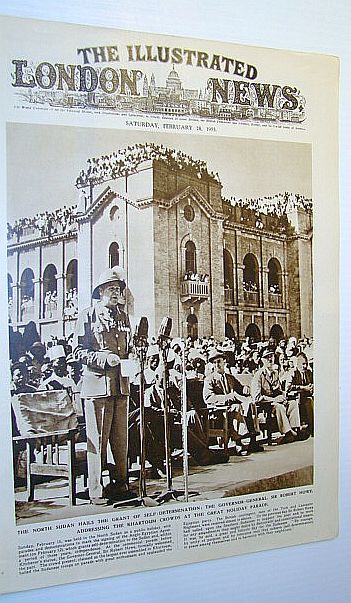This image is an old school poster hanging on a white wall, rendered in a low-resolution, blurred quality. The poster, appearing yellowed with age, is dated Saturday, February 14th, 1921, and is titled "The Illustrated London News" at the top. Dominating the image is a scene outside a large, palace-type building. The structure is teeming with people—packed shoulder to shoulder—on its rooftops, balconies, and around its windows and doors. In the foreground, a man in a military uniform stands on a stage before three large microphones, addressing the crowd. Rows of people, including some black individuals, sit and stand behind him and to his right. Beneath the image, there is a column of text resembling a news story, though it is too small to read clearly.